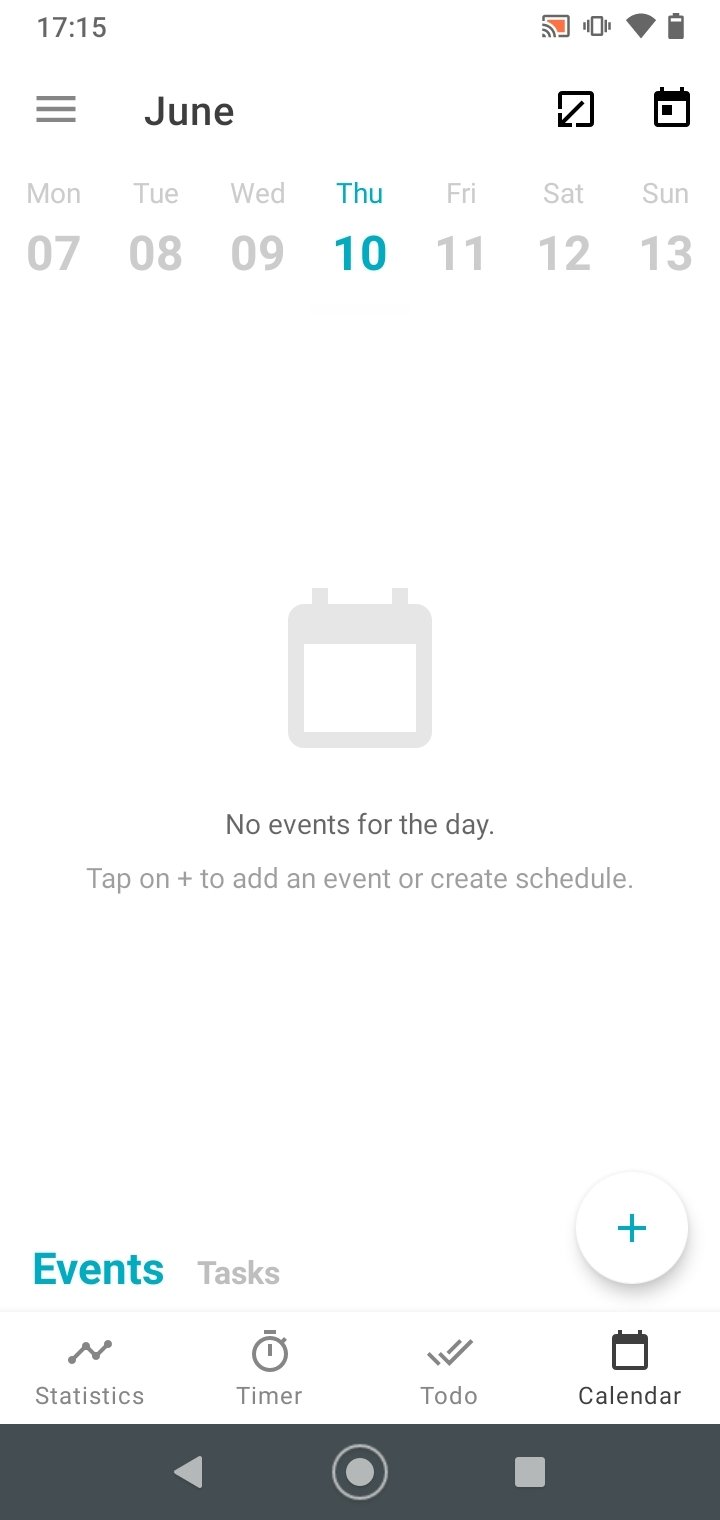A detailed screenshot from a smartphone displays a calendar app against a white background. At the very top, the status bar shows the current time, battery level, and Wi-Fi signal. In the left corner, there is a hamburger menu icon, while the title "June" is prominently displayed.

The current week's dates are listed horizontally, starting from Monday the 7th to Tuesday the 8th, with Thursday the 10th highlighted in blue. Below this date bar, the calendar indicates "No events for the day" accompanied by a small calendar icon and a prompt suggesting to "Tap on plus to add an event or create a schedule."

At the bottom of the screen, there are two tabs: "Events" highlighted in blue and "Tasks" in gray, which likely allows the user to switch between different views. To the right, a blue circular plus button is visible for adding new entries. Below this button are icons labeled "Statistics," "Timer," "To-do," and "Calendar," each with corresponding visuals.

Finally, a dark gray navigation bar spans the bottom, featuring three icons: a back arrow on the left, a circle within a circle in the center, and a square to the right, likely representing common navigation controls (back, home, and recent apps).